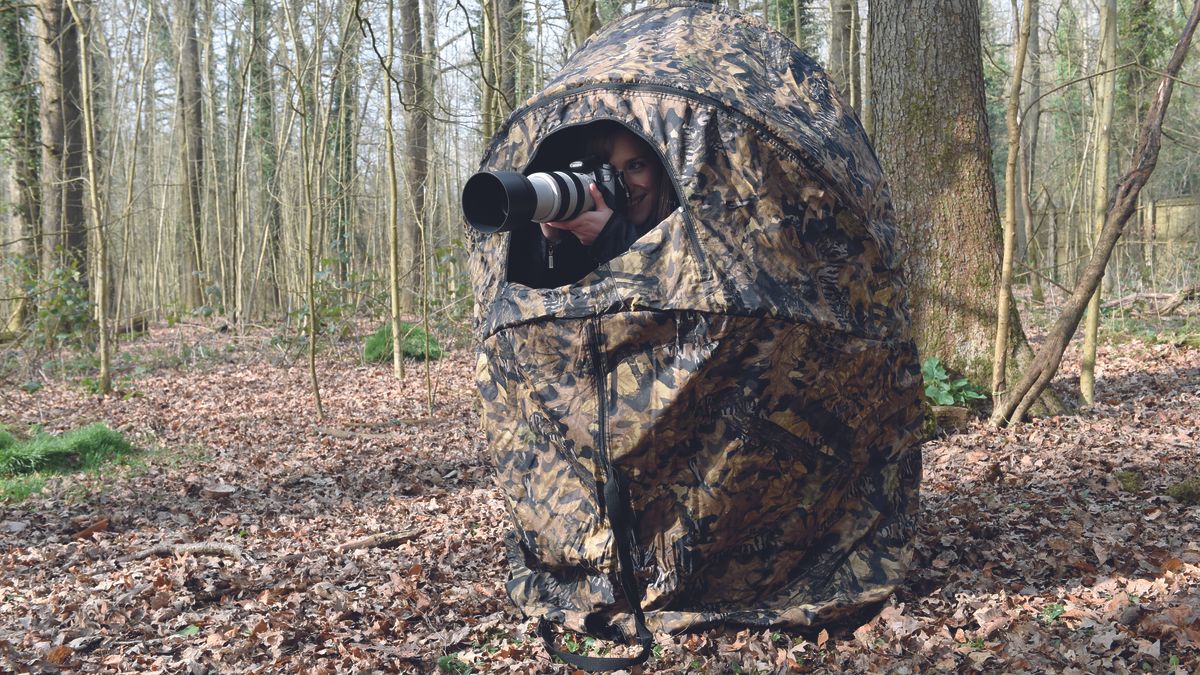In the photograph, a young white woman is nestled within a portable, cylindrical deer stand made from a collapsible ring framework, covered in a camouflage pattern of gray, tan, black, and brown. The deer stand features a small, semicircular window at the top front through which the woman peers while holding a large, sophisticated camera with a telescope lens. She is smiling as she appears to be capturing shots of the natural surroundings. The ground around her is littered with dead leaves, suggesting an autumn or winter setting. The background reveals numerous tree trunks of varying sizes, mostly barren but with some having small green patches. The scene is bathed in sunlight, with hints of blue sky visible through the sparse branches. This clever camouflage setup allows her to blend seamlessly into the wooded environment, making her almost invisible to wildlife as she photographs nature.